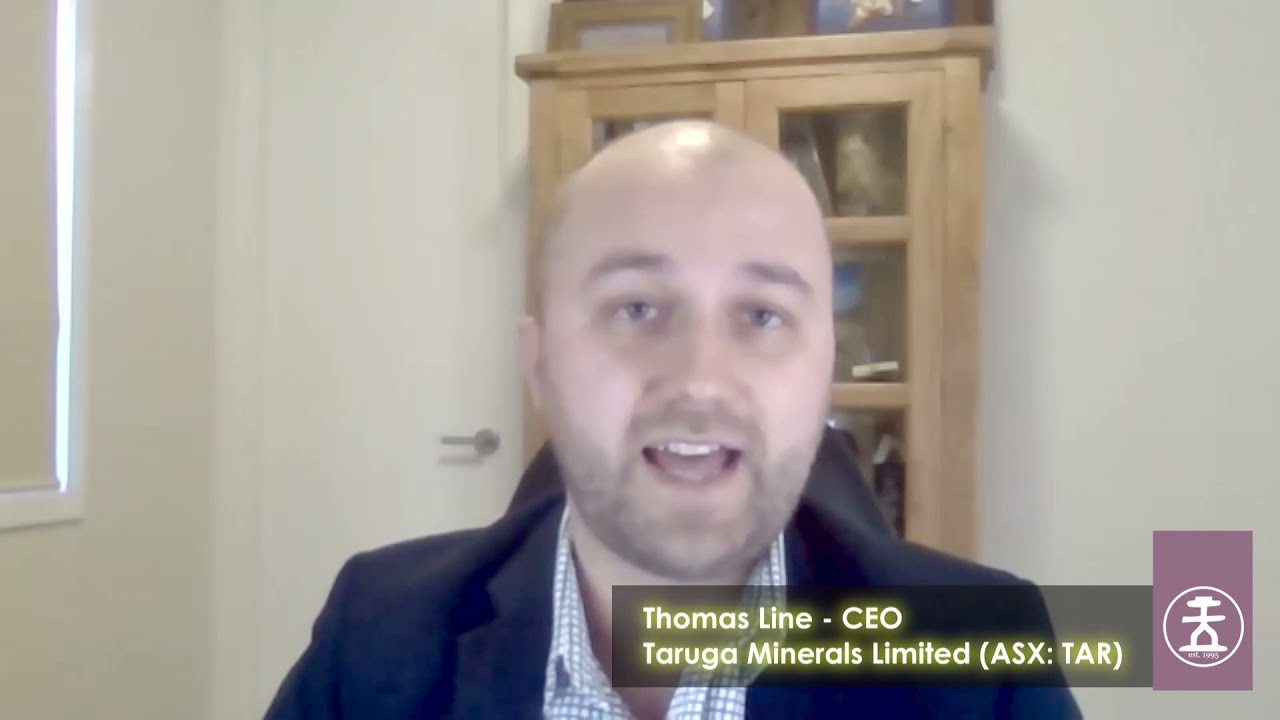In this image, we see a bald white man positioned centrally, looking directly at the camera with his mouth open as if mid-speech. His cherubic face is adorned with thin, black stubble on his cheeks, chin, and mustache. He has light skin, blue eyes, and thin black eyebrows. The man is dressed in a blue blazer over a white, checkered shirt with an unbuttoned collar. He appears to be engaged in a video chat or giving a presentation. He is seated in a black computer chair with a high back. 

Behind the man is a wooden display cabinet with glass doors, containing various objects and pictures. To the left, there's a window with the shade drawn, and to the right of it, a white doorway. The room is well-lit, with off-white, white, black, gray, yellow, purple, and tan colors visible in the setting. At the bottom right of the screen, there is text that reads: "Thomas Line, CEO, Taruga Minerals Limited, ASX TAR," alongside a logo.